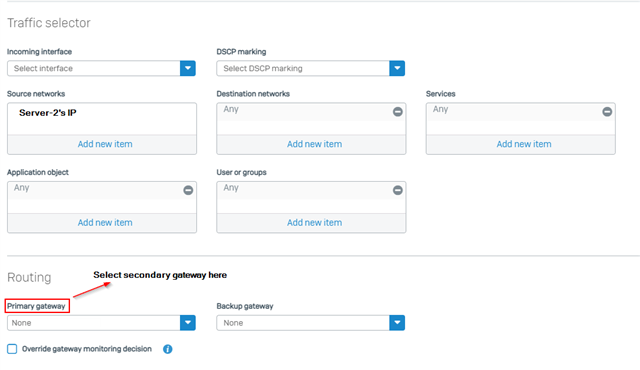**Detailed Descriptive Caption:**

The image showcases a user interface with a blue background and multiple interactive elements. At the top, blue lines frame the main title, which reads "Traffic Selector." Below, the interface features a section labeled "Incoming Interface" with a corresponding dropdown menu embedded within a box. Beneath it, there is an option for "DSCP marking," also accompanied by a dropdown menu.

Further down, the section is divided into various fields: 
- "Source Networks," listing "Server to IP" and an "Add New Item" button 
- "Destination Networks," displaying "Any" and another "Add New Item" button next to a little circle with a line through it
- "Services," again showing "Any" with an "Add New Item" option alongside a blue circle with a white line
- "Application Object" with "Any" and an "Add New Item" button next to the same circle icon
- "User Groups" with "Any" and the "Add New Item" option alongside the same circle icon

Towards the bottom, there is a section to "Select Secondary Gateway," under which routing options are presented. A prominent red box labeled "Privacy Gateways" is highlighted, with a red arrow pointing upwards to the "Select Secondary Gateway" section.

At the lower part of the interface, the settings show:
- "None" under the "Backup Gateway" field
- An option labeled "Override Gateway Monitoring Decision," with a checkbox field and a blue circle containing an 'i' (information) icon next to it.